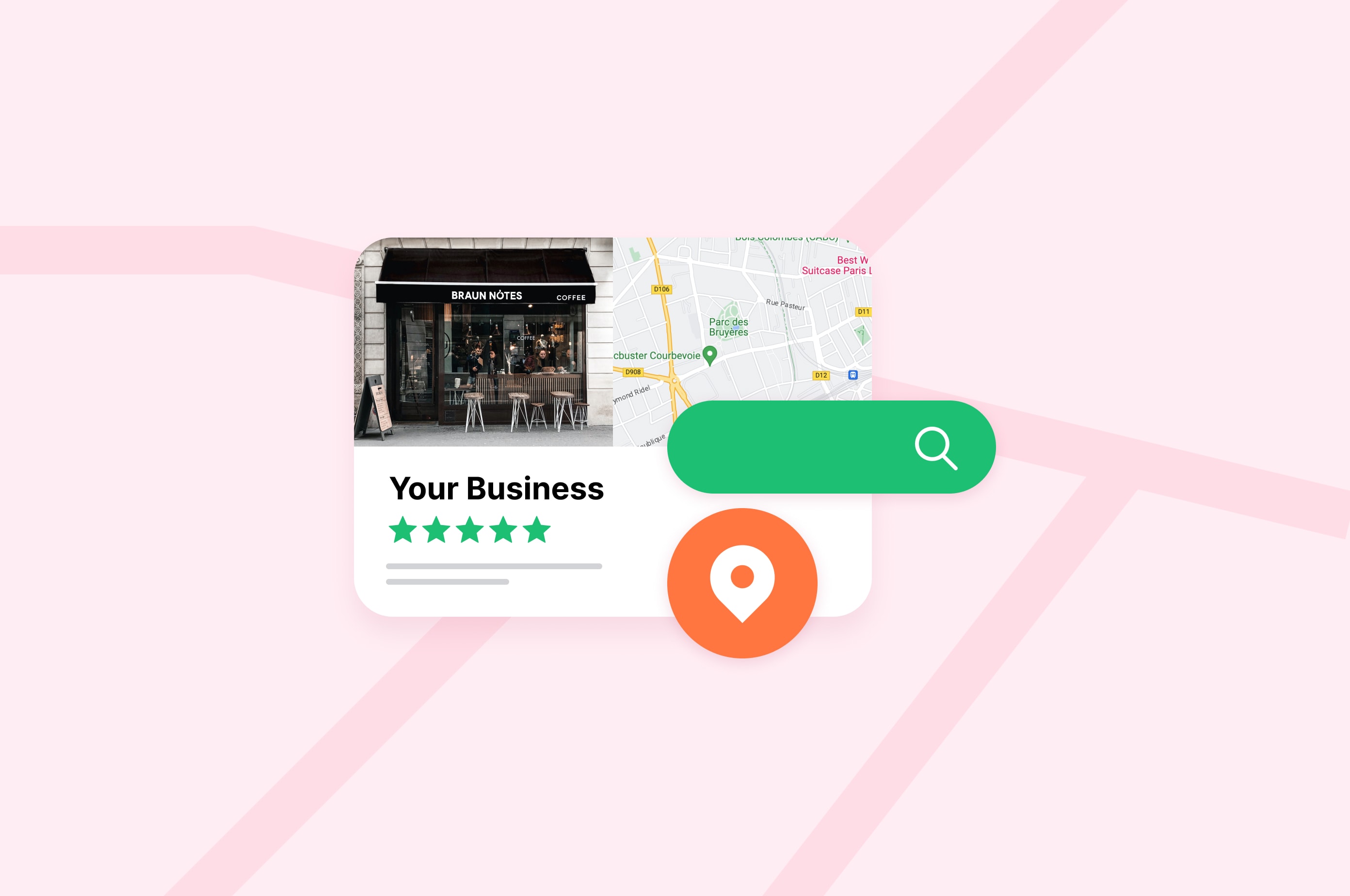This is an image of a Google Maps-like application displaying the location and rating of the "Brown Notes Coffee" shop. The map interface features grey and darker grey roads, with indications of nearby Parisian landmarks, evidenced by French signage and a nearby suitcase company called "Paris." The map includes a green pushpin icon marking the location and a green search bar. The coffee shop has a highly-rated 5-star review, highlighted in the lower left corner with four or five green stars and the label "Your Business." A photo of the cafe's exterior is shown prominently; it features the shop's black-and-white canopy with its logo, providing shade to the outside tables and benches. The cozy atmosphere is enhanced by tables visible indoors through the cafe's windows. Additionally, there's an orange circle with a pushpin icon, likely indicating the precise location of Brown Notes Coffee on the map.